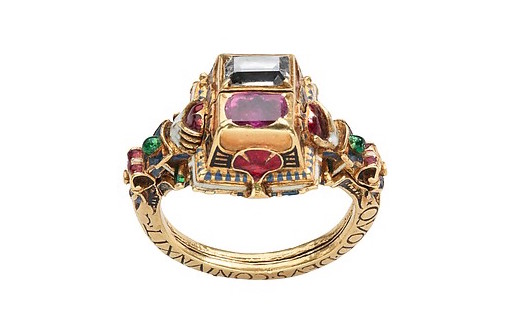The image is a close-up photograph of a very elaborate and ornate gold ring, displayed against a white or transparent background. The band of the ring, which goes under the finger, features an inscription in Latin or a similar classical script, though the text is difficult to decipher and may require turning the ring or image to read fully. 

The ring is adorned with a multitude of colorful gemstones creating a visually striking effect. The top half is encrusted with various jewels, including a prominent emerald-cut gem set within a raised golden square or cube. Below this central stone, likely an amethyst, there are additional gemstones, including potential rubies and emeralds, as well as black and blue stripes that add a touch of an Egyptian motif to the design. The vibrant colors of the stones range from purple and green to red, creating a dazzling and intricate display. The overall craftsmanship of the ring, with its mix of gold and multicolored jewels, gives it an exceptionally rich and luxurious appearance.